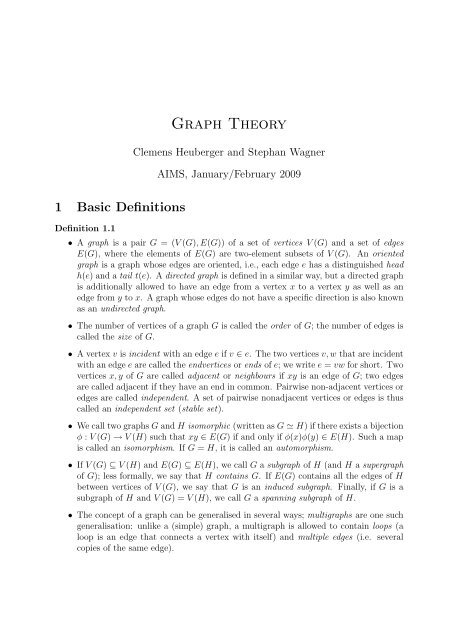The image shows a close-up of a typed page from an academic document titled "GRAPH THEORY." At the top, it lists the authors Clemens, Huberg, and Steven Wagner, along with the date "Ames, January/February 2009." Following the title, the page introduces a section titled "Basic Definitions," specifically denoted as "Definition 1.1." The content consists of approximately six paragraphs, each prefaced with a bullet point and spaced apart for clarity. These paragraphs delve into intricate details of graph theory, starting with a description that states, "A graph is a pair G = (V, E)." Though the print is very tiny and challenging to read in full, the document outlines fundamental terms and concepts, including both directed and undirected graphs, with edges and vertices precisely defined for academic purposes.